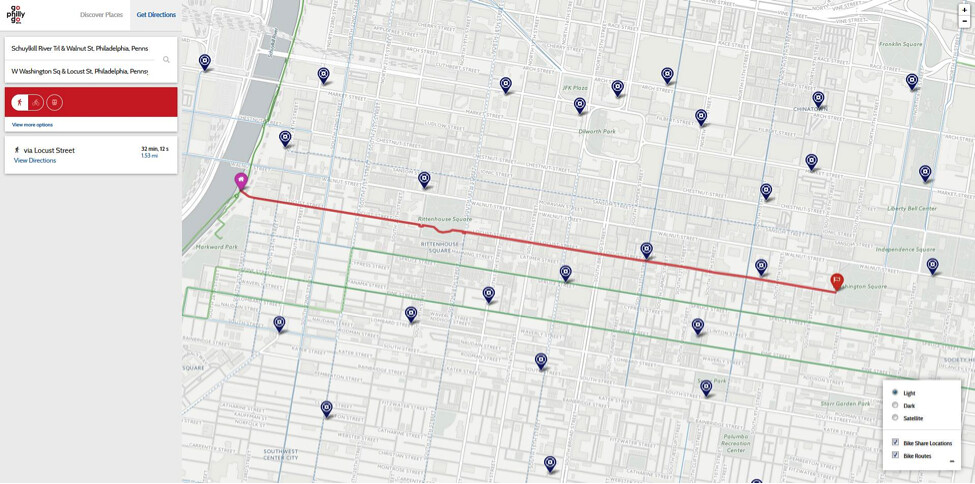This color image features a detailed street map displaying a route from point A to point B. A bold, diagonal line traverses the map from the upper left-hand corner towards the lower right-hand corner, delineating the path in a near-perfect straight line. The journey's starting point is marked by a purple teardrop icon, while the destination is indicated by a red teardrop icon on the right. The map is populated with small blocks, with light gray and light green hues representing different areas.

In the lower right-hand corner, a square legend box provides information about various features, including "light," "dark," "sensitive," "side street locations," and "bike routes." Surrounding the map are small blue teardrop icons, each featuring a solid blue background with a white letter in the center.

At the top right-hand corner of the map, the word "Philly" is prominently displayed in bold black letters, with the exclamation "Go" written above and below it. The "Go" consists of a black 'G' and a red 'O.' Beneath this, the phrase "discover places" is written in light gray, followed by "get directions" in light blue.

Below these inscriptions, there is a rectangular section displaying additional street information. In the middle of this section, a red horizontal bar is depicted with icons of a person walking and a bicycle. Below this, the route is labeled "Walking via Locust Street" in black letters, providing further clarity on the navigation path.